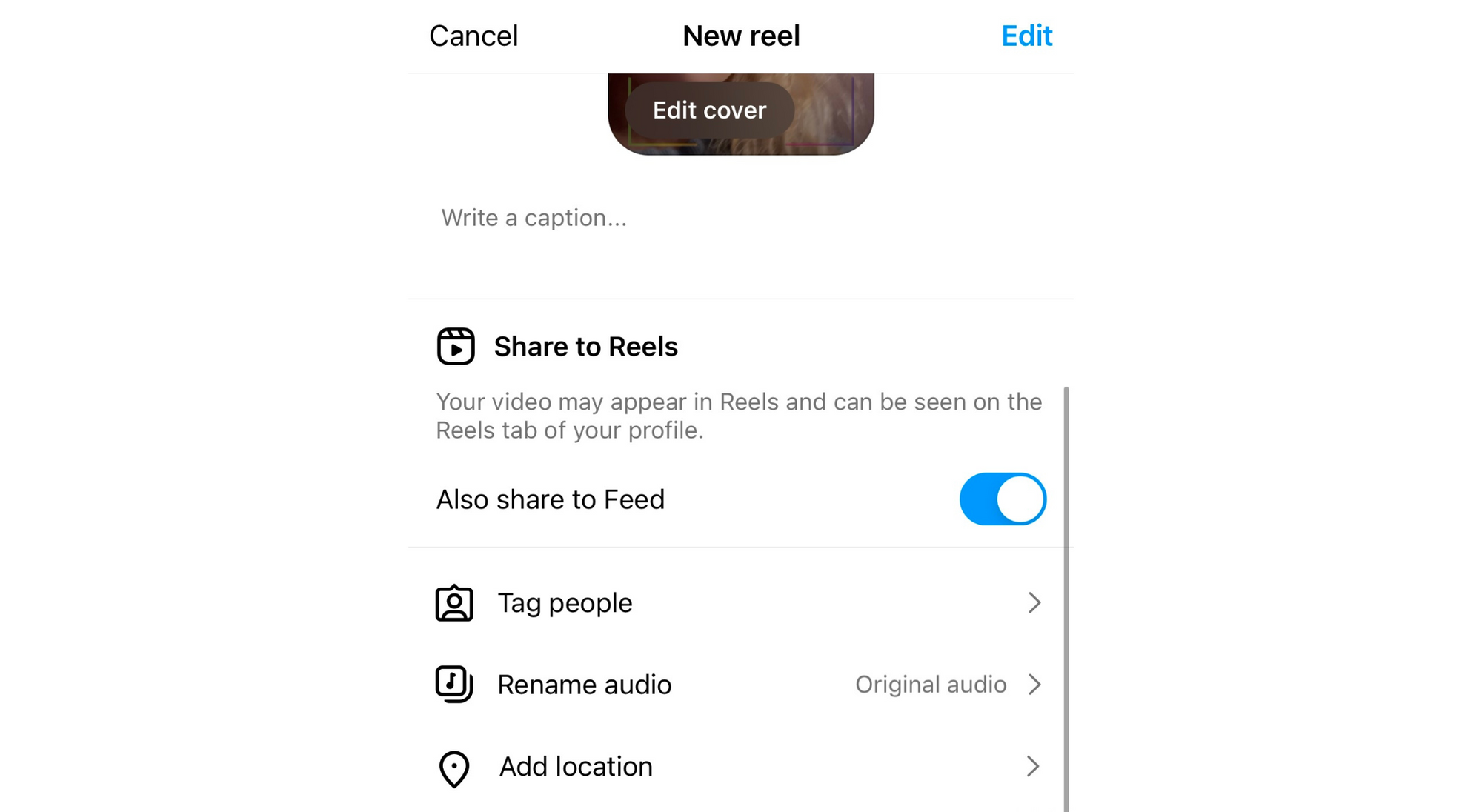This image, likely a screenshot captured from a smartphone, is oriented vertically and showcases a predominantly white background, reminiscent of a computer screen's white display. At the top of the image, on the left, there is a black "Cancel" button, while in the center, the bold black text reads "New Reel." On the right side, a blue "Edit" button is visible. A thin gray line separates this top section from the rest of the image.

Below this line is a partial view of a picture featuring what appears to be swirly brown paint. Overlaying this image is white text that reads "Edit Cover," indicating it can be clicked on.

Further down, there is an option to write a caption, separated by another thin gray line. Below this, a triangle icon signifies a video, accompanied by the text "Share to Reels." The subsequent notification indicates that "Your video may appear in reels and can be seen on the Reels tab of your profile." Additionally, the option "Also share to feed" is enabled, as indicated by a blue toggle switch.

Another thin gray line divides this section from the next, where icons for "Tag People," "Rename Audio" (currently set to "Original Audio"), and "Add Location" are listed, each being clickable options. A final gray line runs vertically down the right-hand side of the image, providing a boundary to the layout.